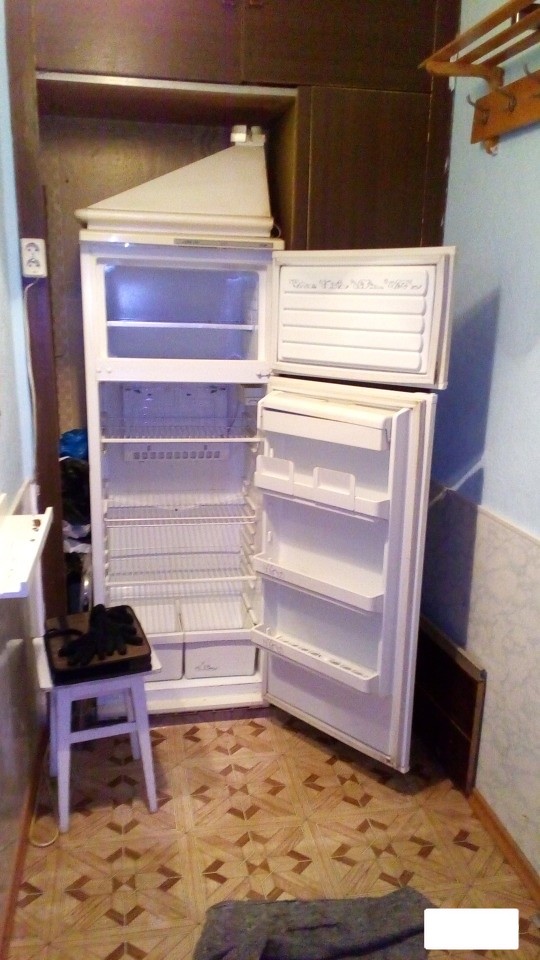The photograph captures a vintage white refrigerator with its doors open, revealing an empty interior comprised of a single shelf in the freezer section on top and two shelves along with some drawers in the refrigerator section below. The refrigerator door has four additional shelves. Positioned in a recessed cabinet-like nook of dark, aged wood, the refrigerator is set amidst a backdrop of eclectic decor. The surrounding floor is tiled with tan and brown linoleum that mimics wood. To the right, a blue wall features a light wood coat hanger with hooks and an outlet that appears to be of European style, along with a vent positioned beneath. In front of the refrigerator stands a small white stool with a brown cushion, and adjacent blue and grey speckled wallpaper adds to the varied texture of the space.